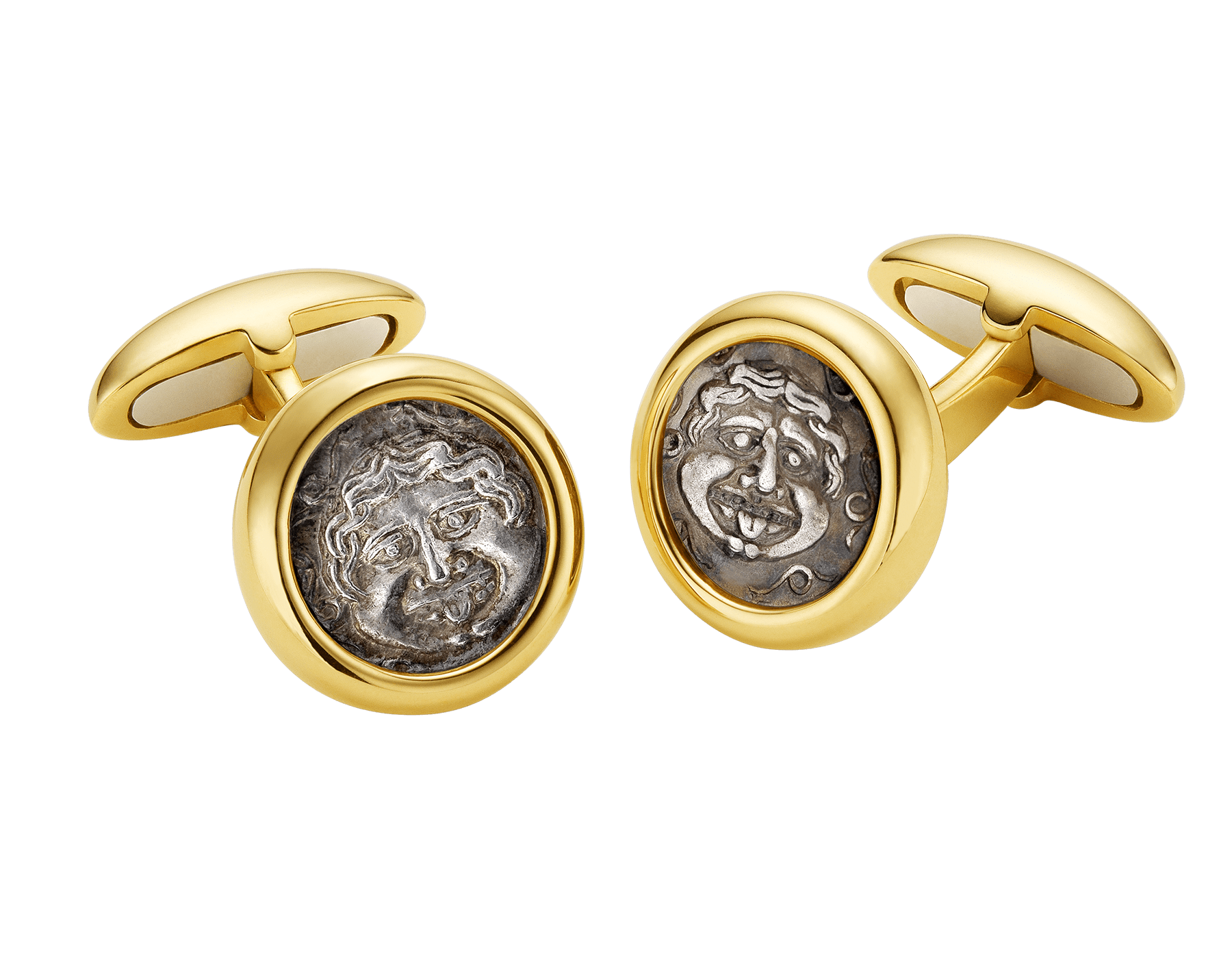This close-up photograph captures a pair of luxurious, designer gold cufflinks placed centrally against a backdrop of pristine white. The cufflinks, characterized by their rich golden rims, feature a distinctive oval-shaped backing, also in gold, connected through a sleek golden tube. The faces of these elegant accessories are adorned with detailed and contrasting silver-hued inscriptions set against a darker grey background, highlighting the unique craftsmanship. Each circular cufflink features two distinct faces: on the left is the face of a man with grey hair, smiling, and on the right, a woman playfully sticking her tongue out, perhaps wearing eyeglasses. The intricate design embodies a blend of sophistication and modernity, making these cufflinks stand out as both functional accessories and pieces of art.